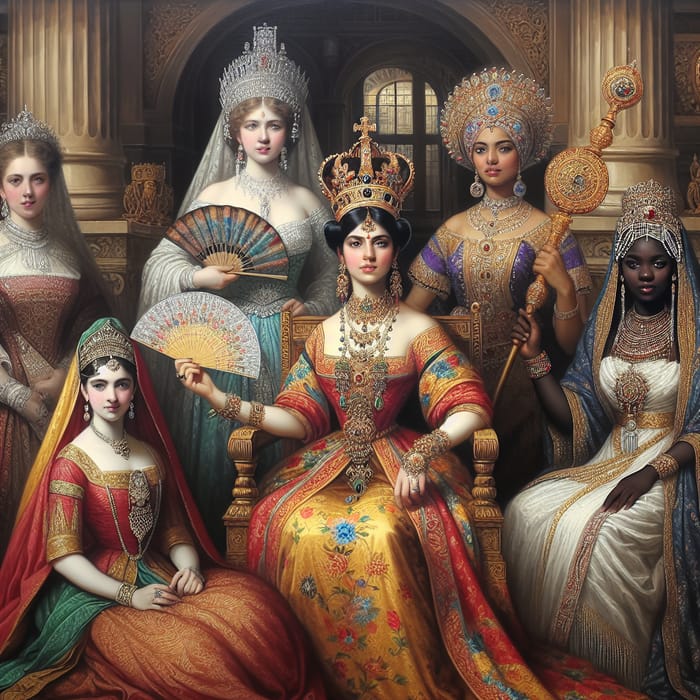This is an intricate illustration of a royal court, portraying a diverse assembly of queens from different regions and ethnicities. At the center sits the principal queen on an ornately carved wooden or golden throne, adorned with a majestic crown featuring a cross on top. Her black hair is elegantly tied up, showcasing a forehead dot and elaborate forehead jewelry. She wears a magnificent Indian-style robe in warm hues, embellished with blue flowers, gold earrings, multiple ornate necklaces, and gold wristbands. She holds an intricately designed fan in her right hand.

Surrounding the central queen are five other regal women, each adorned in luxurious gowns and elaborate jewelry, but with less opulence compared to the main queen. To the immediate right and left of the queen are two Indian-looking queens, one in a more African-inspired outfit. Behind them, two fair-skinned queens stand, one possibly Russian with a diamond crown, and another with blonde hair. Each has a distinctive style, reflecting their diverse heritage.

To the far right stands a striking black queen in a contrasting white gown, adorned with pearls and silver jeweled drapings over her forehead. Every queen is crowned, some holding symbols of power such as a golden staff. They are positioned against a backdrop of classical style columns and an arched window, adding to the grandeur of this royal assembly. All the women, despite their diverse backgrounds, share a solemn yet welcoming expression, capturing the elegance and unity of this royal depiction.